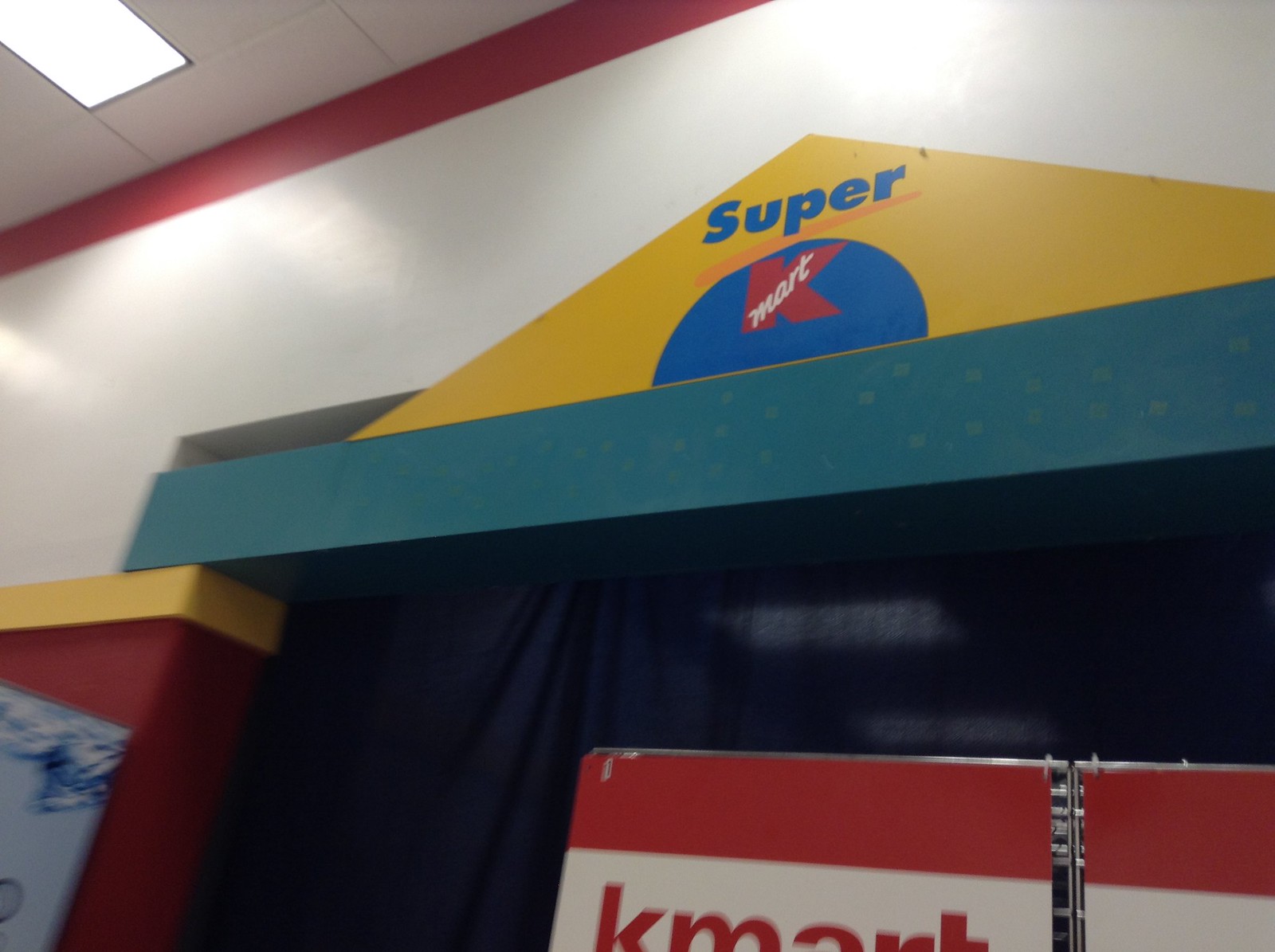This photograph captures an indoor section of a Super Kmart store, focusing upward toward the ceiling. The image features a white wall with an archway-like cutout, above which is a lighter blue crossbeam. Draped over this cutout is a navy blue shade or curtain. Prominently displayed above the archway is the Super Kmart logo, comprised of a yellow triangle with "Super" in blue text and a red "K" with white "mart" script against a blue half-moon shape. Below this, visible through the semi-transparent shade, are two fluorescent ceiling lights. The ceiling itself consists of acoustic tiles with inset lights and a red trim running along the top edge. To the left-hand side of the frame, there is a red wall adorned with a yellow trim and another Kmart sign in red letters against a white backdrop.